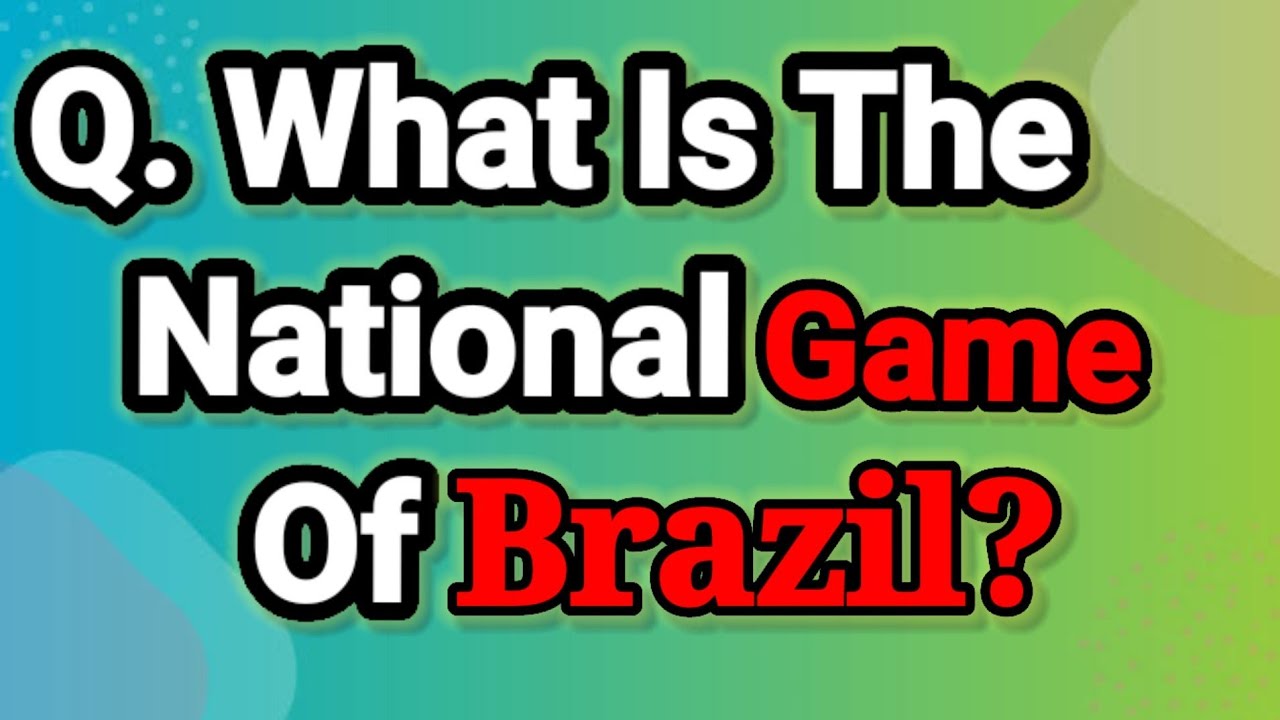In this vibrant and colorful website layout, the left side is dominated by soothing shades of blue, while the right side showcases various shades of green. An image of a light green box occupies the upper right-hand corner, and a light blue box image is positioned in the lower left-hand corner. 

The centerpiece of the website features a prominent question presented in bold, eye-catching text. The header starts with "Q dot" (short for question), encircled by blue dots. The main question text is displayed in large white letters with a thick black outline, making it easily readable. The unique typography features curved T's at the base, adding a distinct touch. The question reads, "What is the national game of Brazil?" in a combination of red, black, and white text, ending with a striking red question mark next to the word "Brazil."

Despite its visually striking presentation, the origin of this webpage remains unknown, and it provides no clear instructions or links on where to find the answer to the posed question.